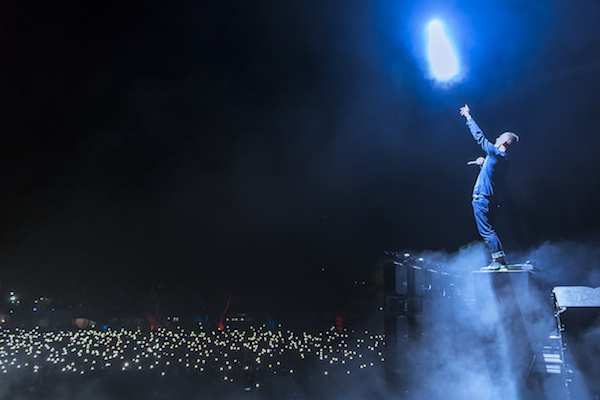The image depicts a blurry, horizontally aligned rectangular picture of a male singer on stage, captured from a side view. He is positioned on the center-right side of the image, wearing an all-blue outfit consisting of a blue jacket and blue pants, with short brown hair. His left arm is extended upward towards a bright, white ceiling light that creates a streak of illumination, while his right hand, which seems to be holding a microphone, is stretched out to his side. The stage is enveloped in fog, adding to the atmospheric mood. The background is solid black, enhancing the glow of numerous lit candles or phones held by the audience, which are clustered densely, especially in the lower left corner of the picture and spread out towards the lower right. The sea of flickering lights emphasizes the concert’s nocturnal setting, creating a mesmerizing contrast with the solitary, brightly lit performer on stage.